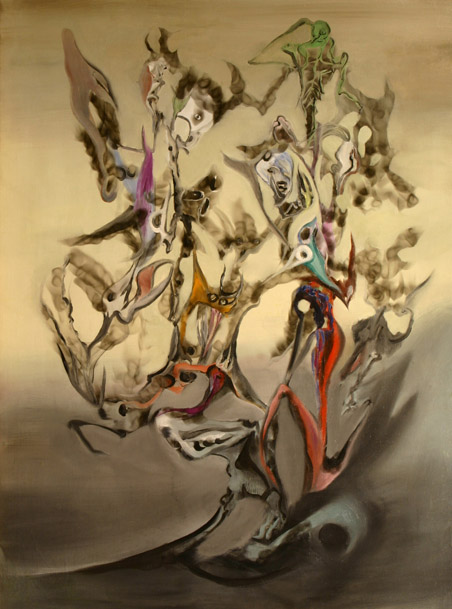The painting is a captivating abstract piece, set against a dark yellowish-brown background that deepens toward the bottom. Dominated by flowing, flame-like shapes emanating from a half-buried, broken animal skull at the base of the composition, it evokes the release of haunting entities. Among the swirling mist and colored forms—ranging from reds, yellows, greens, and purples to teals—various blurred faces and outlines appear. There's a haunting green skeletal figure near the top right, an equine-like face, horned animals, and even a bird, all blending seamlessly within the brown mist. The mixture of shapes and colors creates a dynamic, evocative scene with no definitive forms, emphasizing the ethereal and haunting quality of the image.